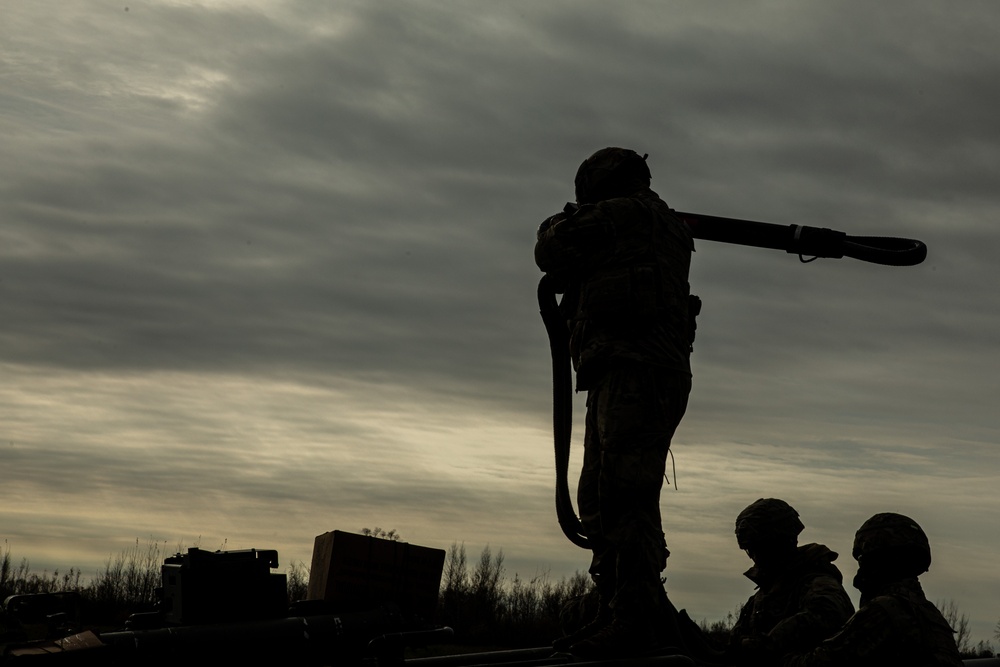In this dark, brooding grayscale image, three soldiers are captured amidst a wartime scene. The dense, overcast sky transitions through shades of gray, with mottled patches from light to dark, and doesn't permit much light through, creating a shadowy, ominous atmosphere that feels like late evening or nightfall. In the foreground, blackened grass stretches across the bottom, and an ammo box is nestled within it. The feet of one soldier, who is standing, are visible—this soldier has a large weapon mounted on his shoulder, likely a rocket launcher, with something draping down from it. Although his form is shadowy, his position is prominent, slightly to the right of center, and he appears hunched over, aiming the weapon. Below him, as if in a trench, the heads and shoulder portions of two other soldiers are seen, their helmets discernible against the murky backdrop. The overall scene carries a tense, shadow-heavy ambiance, intensified by the indistinct dark shadows of distant foliage to the left, likely grass or trees. The soldiers’ army gear blends into their silhouettes, presenting a stark, ghostlike presence in this somber setting.